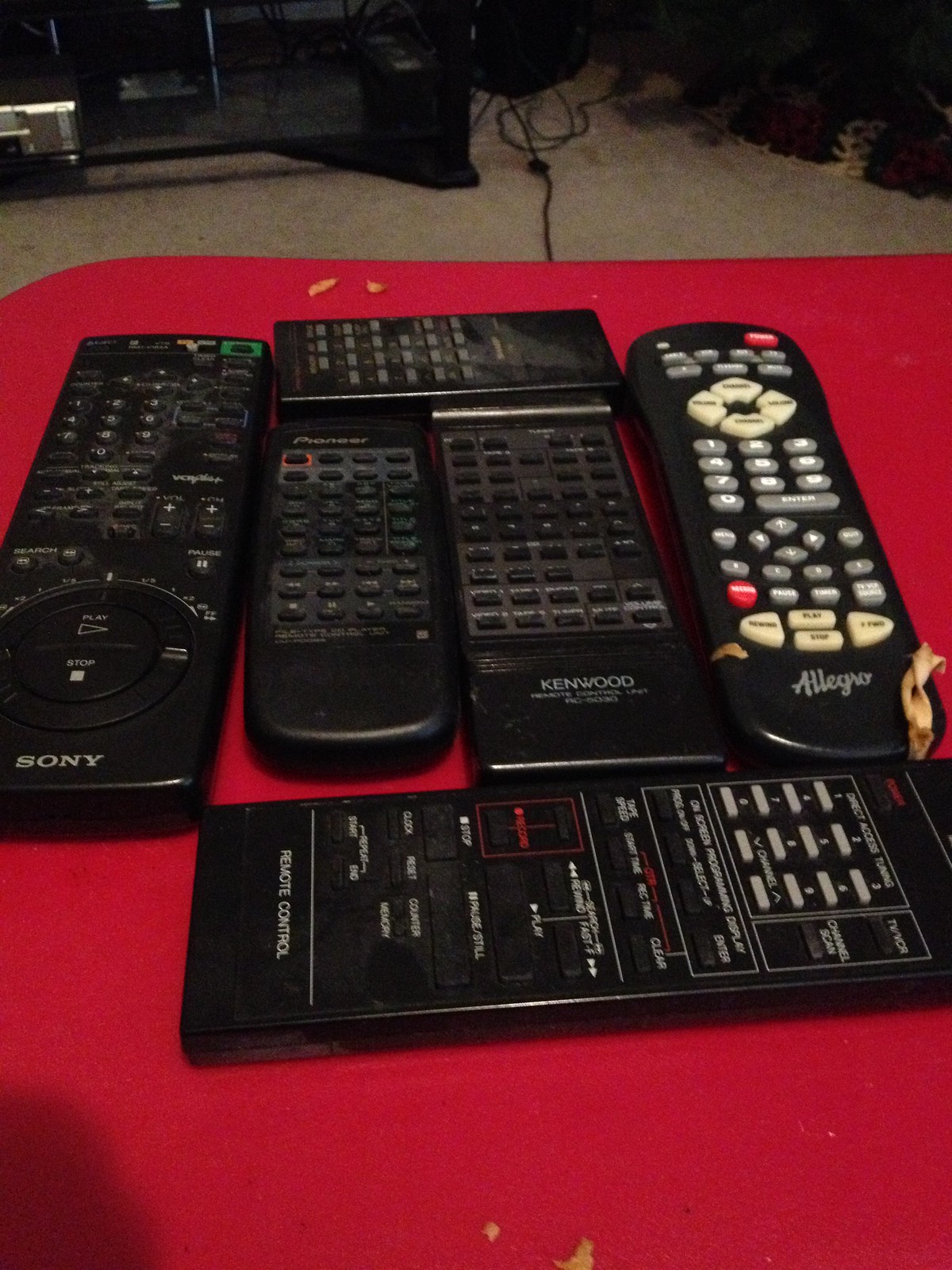The image is a color photograph of a variety of old, dusty remote controls arranged on what appears to be a red, padded tabletop with visible tears exposing foam underneath. Several remote controls of different brands, including Sony, Panasonic, Kenwood, and Allegro, are scattered across the table, each displaying signs of wear. Notably, the Allegro remote has white and gray buttons and is held together by a thick rubber band to secure the battery cover. Among the other remotes, one is shaped like a smartphone but is not a TV remote, hinting at its function for controlling a different type of device. In the background, a beige carpet and a piece of what looks like an entertainment console with trailing electrical wires can be seen.